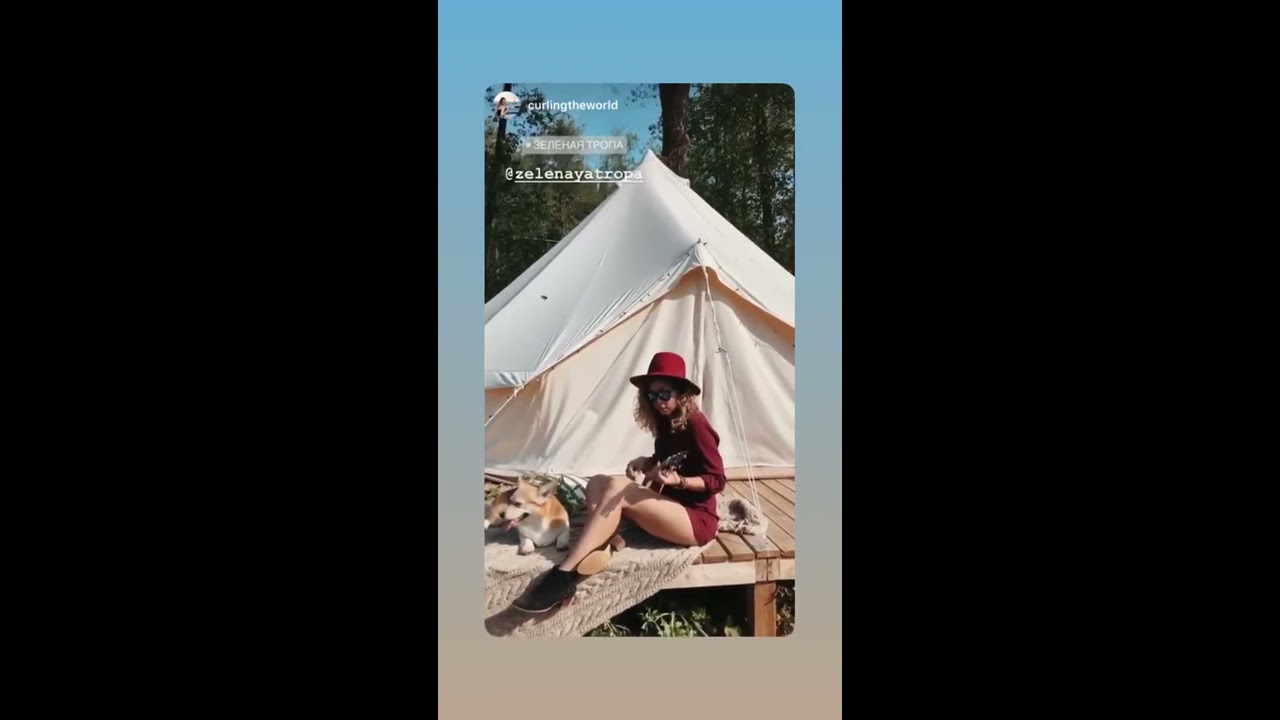The image appears to be a screen capture from someone's social media page, presented with thick black borders on both sides, creating a narrow vertical frame for the central photo. The image itself showcases a young woman with curly blonde hair, sitting on a light brown wooden deck that is slightly elevated with visible support poles beneath it and grass below. She is dressed in a dark crimson red, very short dress, paired with a matching crimson red hat and black shoes. She sits in front of a cream-colored fabric tent, holding a guitar and facing to the left. Her legs are prominently visible from the hips down.

In the bottom left corner of the deck, partially covered by a cream-colored blanket, sits a small tan-colored dog, possibly a corgi, with its mouth open and tongue out, facing left. The backdrop to this scene includes several trees with green leaves. At the top of the image, there is white text that reads "Curling the World" and the handle "@ZelinaTropa," accompanied by a small circular avatar, presumably of the woman. The image is framed by a border that shifts from light blue at the top to a grayish color at the bottom.